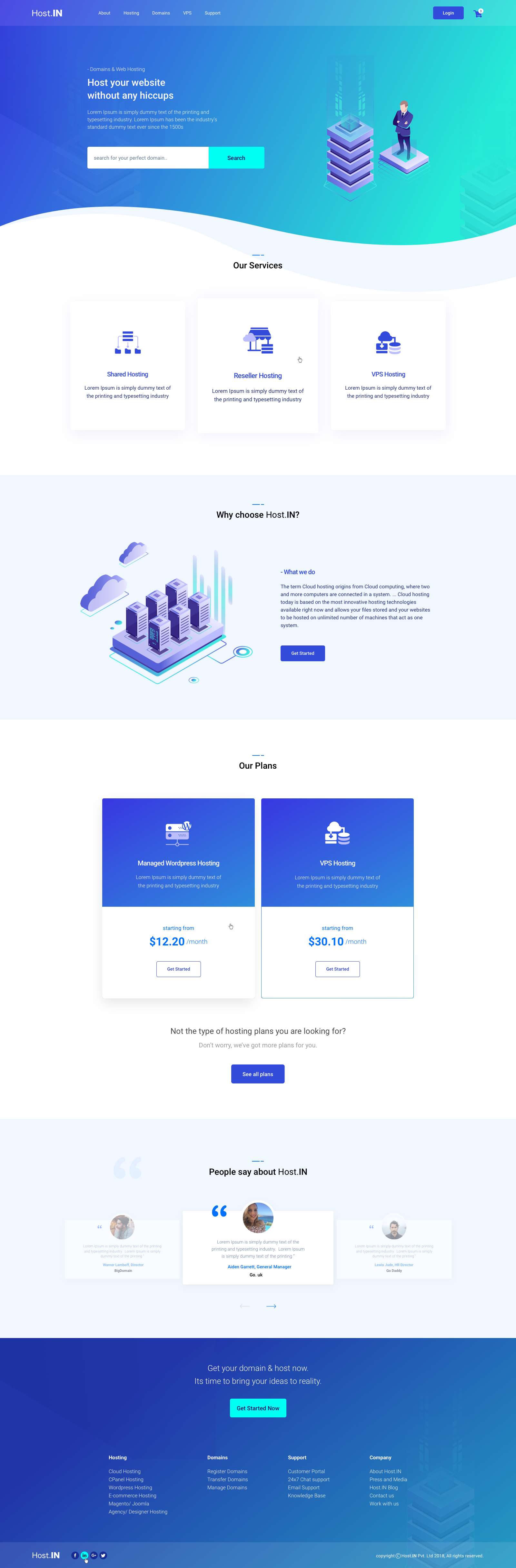**Caption:**

The web page depicted in the image is styled using a sophisticated palette of dark blue, white, black, gray, and bright turquoise blue. In the upper left-hand corner, the word "host." is displayed in white stylized text, followed by "in" in bold. To the right of this stylized text are clickable white text links for hosting, domains, VPS, and support services. On the far right end of the navigation bar, a dark blue rectangular button with rounded edges and white text reads "Login." Adjacent to this button is a blue shopping cart icon with a white circle overlay, displaying the number "3" in black.

The webpage's main body features prominent white text proclaiming "Host your website without any hiccups, domains, and web hosting." To the right of this phrase is an animated illustration of a man with light skin and short brown hair, dressed in a navy blue vest, black pants, a black necktie, and a white shirt. He stands on a gray rectangular platform, looking at a stack of lilac, pastel purple, and dark blue square boxes.

Further down the page, under a black header that reads "Our Services," blue text lists various hosting options: shared hosting, reseller hosting, and VPS hosting. Another black header below this section reads "Why choose host.in," followed by blue text stating "What we do." This is accompanied by a pastel purple, navy blue, and turquoise illustration of clouds and small rectangular nubs on a larger flat surface.

The final section includes a black header titled "Our Plans," under which two blue boxes with white text offer "Managed WordPress Hosting" and "VPS Hosting." Pricing details are provided below, with text indicating "12.20/month" and "30.10/month," respectively.